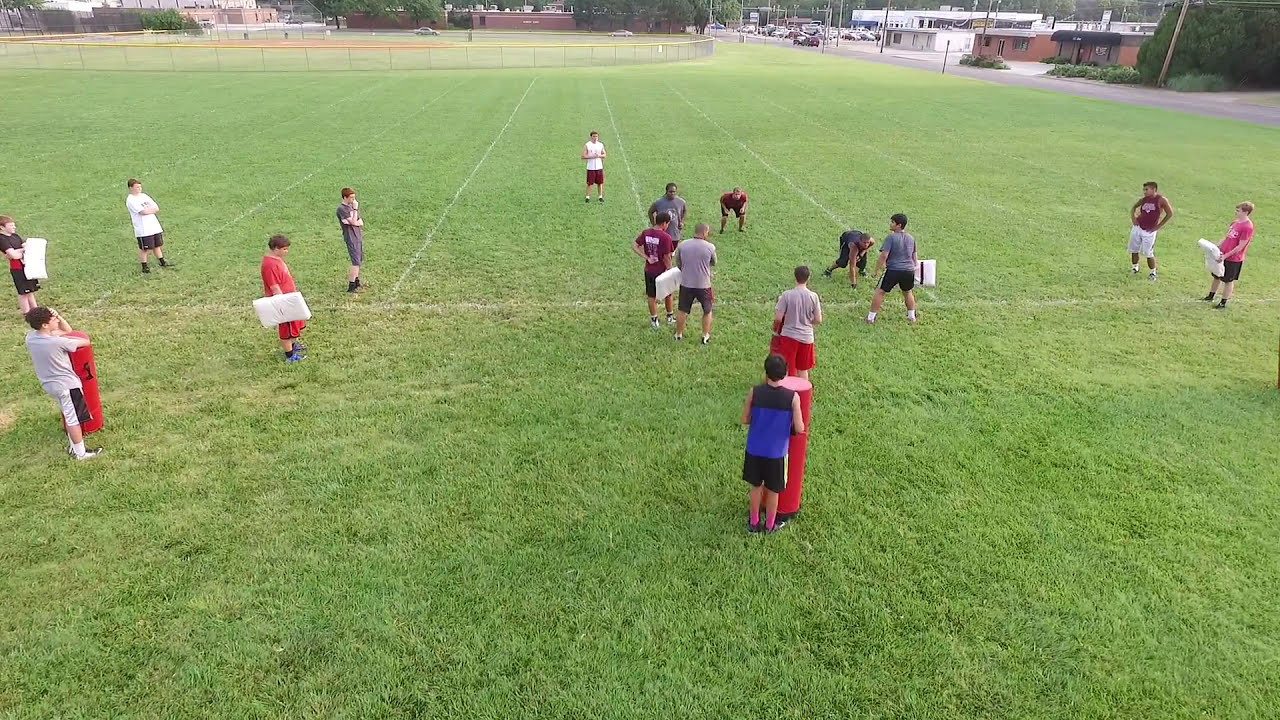The photograph captures a group of approximately 15 to 20 boys, aged around 12 to 14, engaged in some form of athletic drill on a somewhat worn green turf field. The field features chalk-drawn rectangles forming distinct rows and columns. The boys are dressed in casual shorts and t-shirts, indicating a warm day. Scattered among them are several white cylindrical mats and rectangular pads, commonly used in defensive football drills, along with a few orange cone markers. In the center of the gathering, a few adults of diverse racial backgrounds appear to be discussing the activities. The field itself is not well-maintained, with visible dark patches interspersed among the greener areas. Beyond the field, a road and a fence are seen, alongside other sports fields and possibly school buildings. The scene suggests a casual yet organized sports practice, likely football, given the equipment and setup.